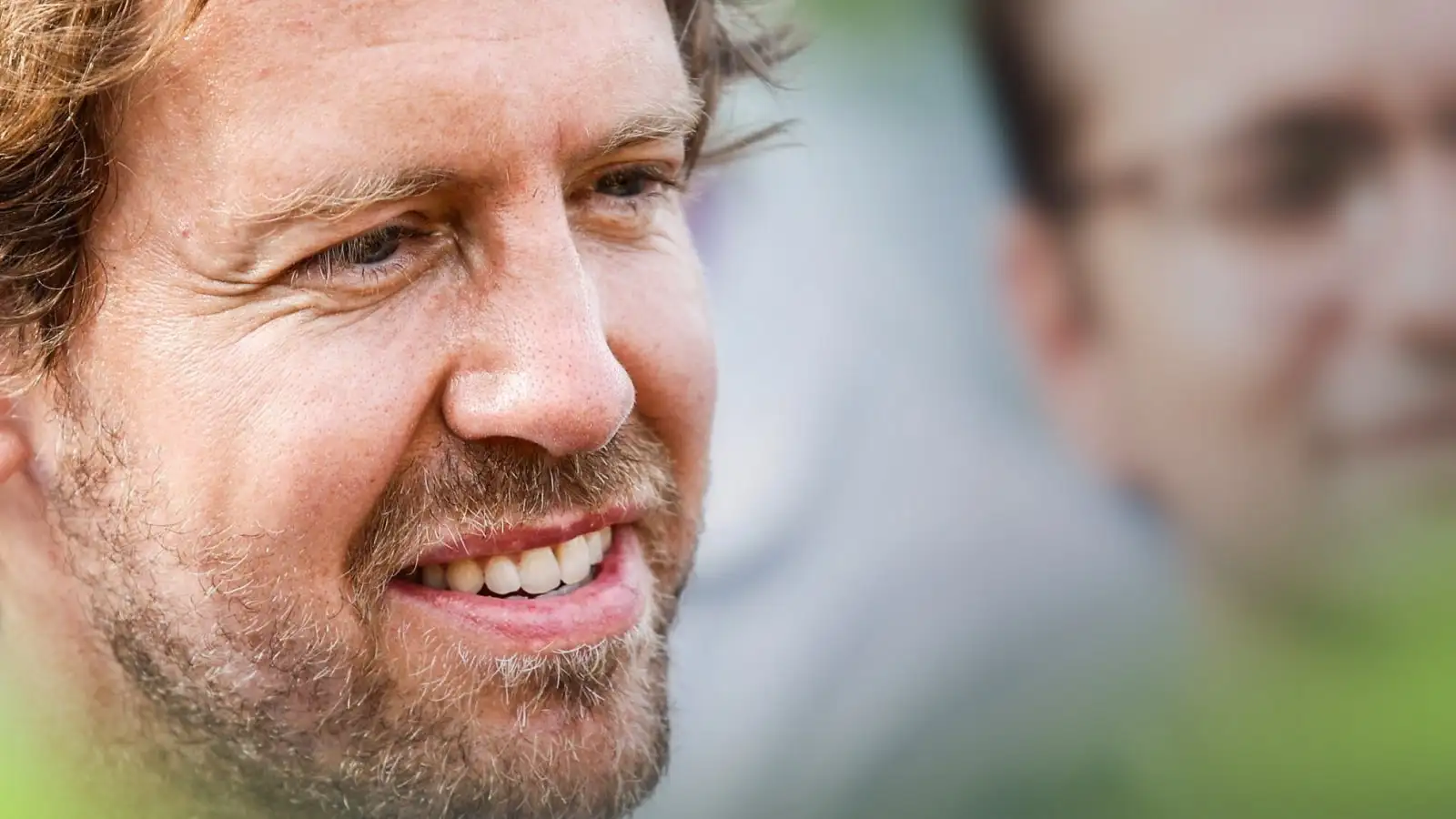This photograph features a middle-aged man with brown hair and a scruffy beard speckled with gray, occupying the left half of the image. His face, filling the frame, is detailed with wrinkles around his eyes, hinting at his age. The man gazes slightly downwards to his right, his gentle smile revealing his upper teeth. In the background, slightly out of focus, is another man with short brown hair and glasses. He, too, wears a faint smile, and only a portion of his face, including his ear, is visible. The background is a blurred green, with an indeterminate object in the lower right corner of the frame.